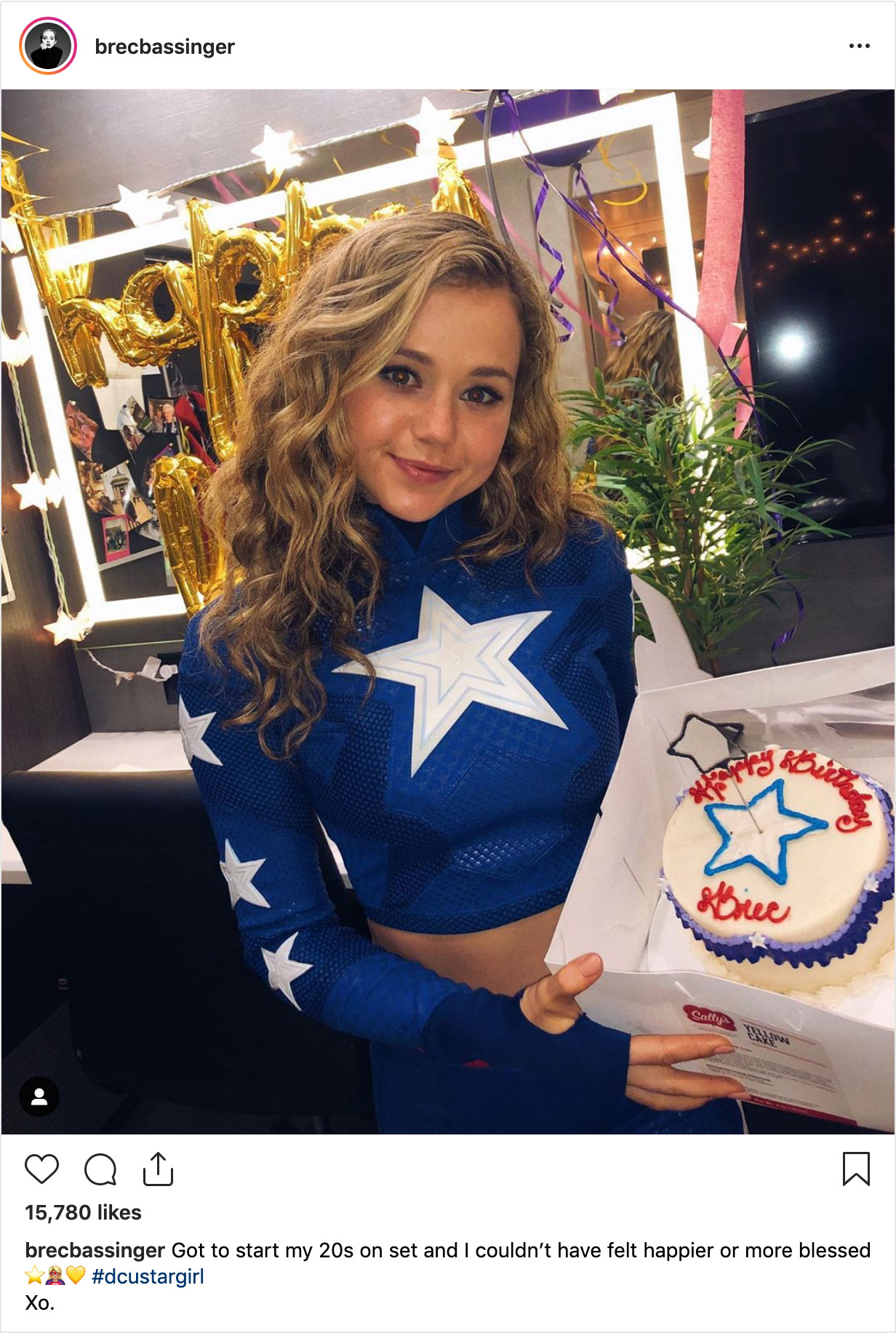In the image, Breck Basinger, dressed in her Dallas Cowboys cheerleading uniform featuring a blue star on her left sleeve, is holding a white birthday cake adorned with a blue star in the center and decorative blue swirls around the edges. The cake, from Sally's, bears a difficult-to-read cursive message that says "Happy Birthday Brie." Breck, a young woman with long, curly blonde hair, stands in a room decorated with a "Happy Birthday" sign, smiling directly at the camera. Her Instagram post, which has garnered 15,780 likes, includes the caption: "Got to start my 20s on set and I couldn't have felt happier or more blessed. XO, Star Girl 💫."